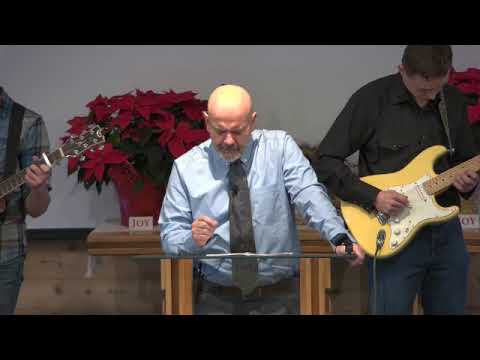The photograph captures a solemn church scene with a central figure standing at a pulpit. This man, of Caucasian descent, is bald with a gray beard and dressed in a long-sleeved, button-up blue shirt, a black tie, and gray jeans. His eyes are closed, and his brow is furrowed, suggesting he's deeply engaged, possibly in prayer or in delivering a sermon. To his left stands a man partially visible, holding a guitar, while to his right, another Caucasian man with his head bent down is actively playing a yellow guitar. This second guitarist is clad in a black, long-sleeved, button-up shirt and blue jeans. Behind the central figure is a prominent display of red poinsettia plants, creating a festive backdrop. In front of the poinsettias, a white card with red lettering bears the word "Joy," adding a celebratory note to the scene. The overall setting is casual yet reverent, indicating a church environment where music and worship are integral elements of the service.